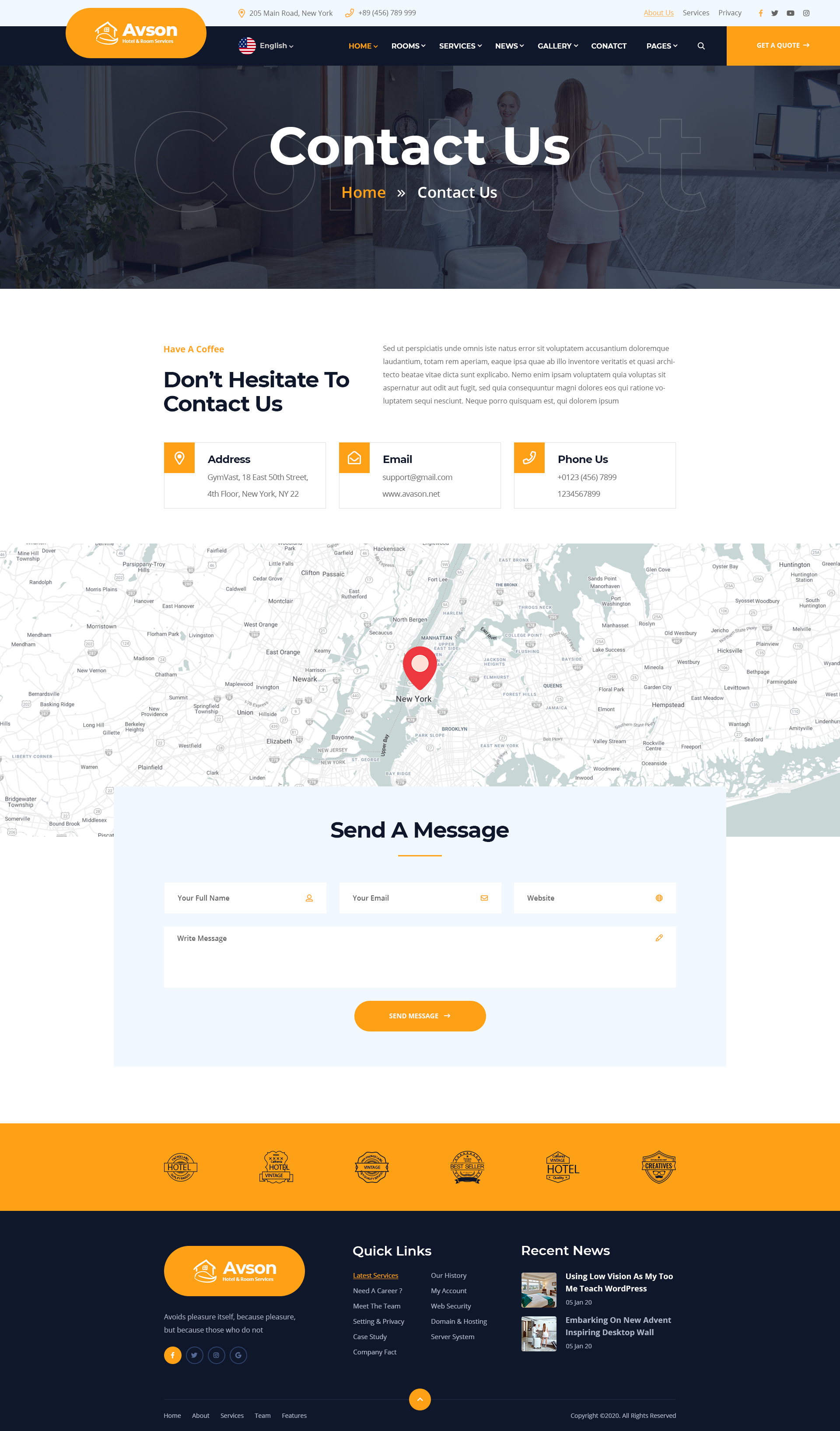This detailed screenshot captures the interface of a webpage for ABSON Hotel and Room Services, located at 205 Main Road, New York. The top of the page features a gray bar with navigation options including About Us, Services, and Privacy. In the top left corner, there's a yellow oval logo with a house and leaf icon, labeled "ABSON."

The header menu allows users to navigate to Home, Rooms, Services, News, Gallery, Contact, Prices, and Get a Quote. The central part of the screenshot features a photograph of three people conversing in a room, overlaid with a dark gray or blue tint. Overlay text reads "Contact Us" and "Have a Coffee, Don't Hesitate to Contact Us."

Below this, a placeholder paragraph in Latin is displayed, implying future content. The contact information provided includes the address of Jim Vest at 18 East 50th Street, 4th Floor, New York, NY 10022, email support at gmail.com, website www.abson.net, and a phone number +89-456-789-999.

To the right, a map of the New York metro area is shown, accompanied by a contact form titled "Send a Message," asking for Full Name, Email, Website, and Message, with a button to submit the form entitled "Send a Message."